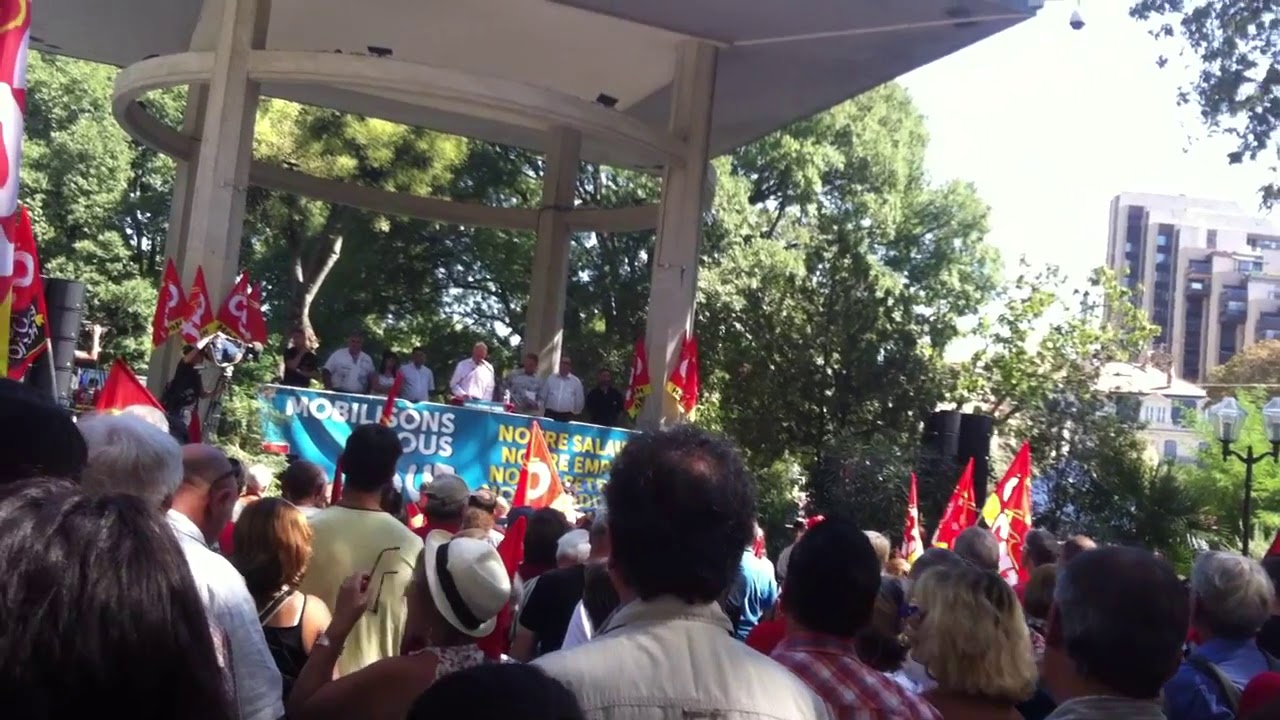This photograph captures a vibrant political rally set in an outdoor park, centered around a pavilion or kiosk. In the foreground, a large crowd is gathered, consisting of an uncountable number of people whose heads form a sea directed towards a raised platform. The scene is bathed in sunlight, enhancing the lush greenery of the tall trees that form the backdrop. 

Prominently displayed on the pavilion is a banner with partially legible French text, possibly reading "O-U-S-N-M-O-E-I-L-L-O-N-S" or "M-O-B-I-L-S-O-N-S-N-O-S-A-L-A-E-E-M." The banner adds an international element to the rally, indicating it may be a demonstration or protest with significant meaning. Six individuals stand on the platform, addressing the crowd, likely leaders or key speakers of the event.

Red flags are a notable feature, mounted on either side of the pavilion and waved by several people in the audience. These flags have white designs that remain indistinguishable due to their partial display. In the background, behind the pavilion, are tall buildings visible in the far right corner, set against a cloudy sky, further framing the setting as an urban park area. The scene is dynamic and charged with the energy of collective action.